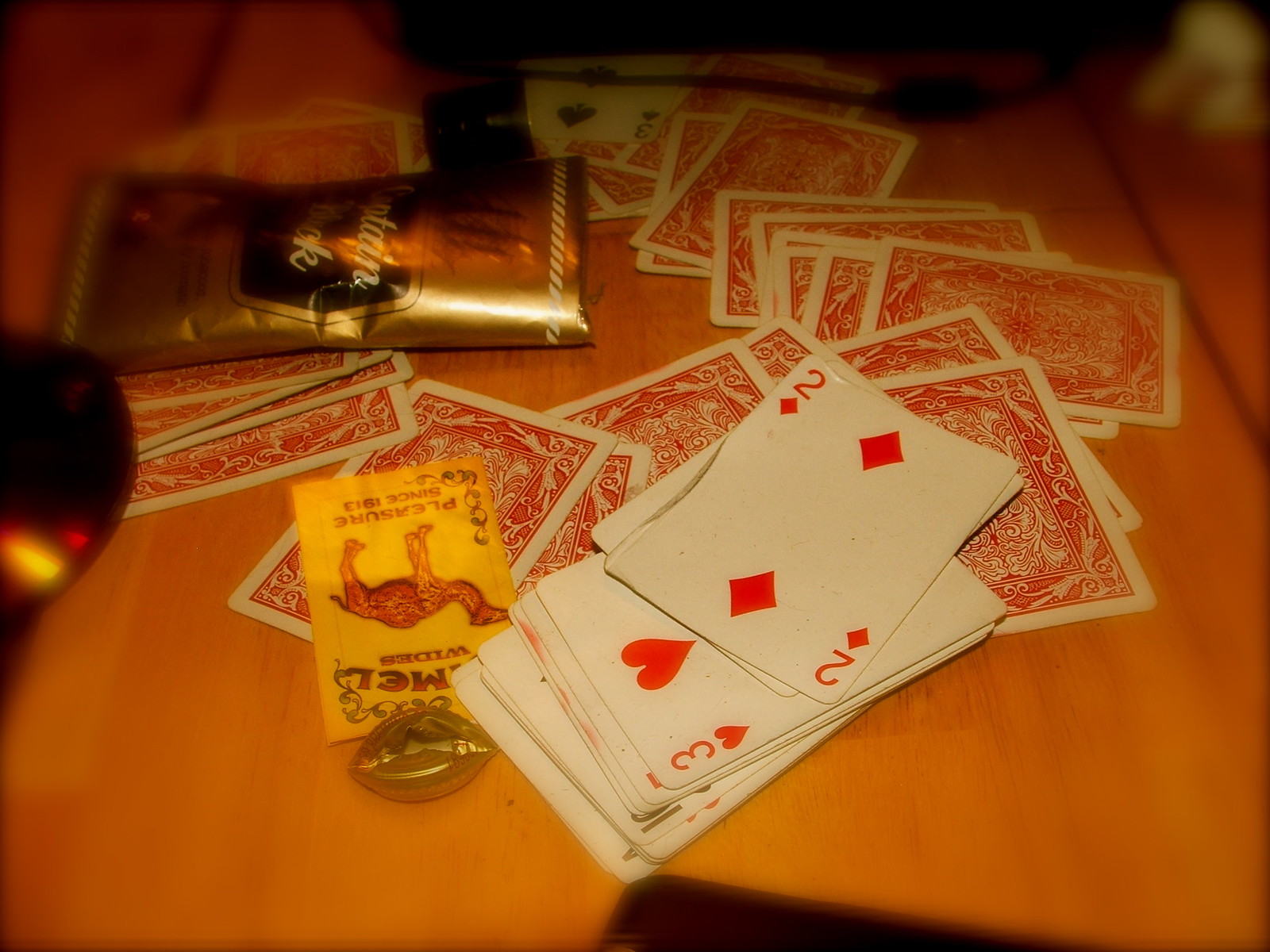In this photograph, a collection of playing cards is spread out across a light brown wooden table, providing a rich and detailed scene. At the lower section of the image, a small stack of face-up cards reveals their fronts. The topmost card is the 3 of hearts, distinguished by a red numeral "3" and a red heart symbol in the opposite corners. Just beneath it is the 2 of diamonds, which displays a red "2" in the corner, complemented by a red diamond shape beneath it and two additional diamonds positioned centrally. Notably, this card shows significant wear, with its lower left side visibly bent and warped.

Surrounding the stack, other cards are dispersed in a circle, their backs facing up. These card backs are characterized by a red background bordered in white, adorned with intricate white shapes and an elegant interwoven pattern in red and white. To the left of the face-up stack sits a rectangular Camel Cigarettes card, seemingly an advertisement. This card features elaborate border designs and bold text.

In the top left corner of the photograph, a silvery plastic package is visible, containing an unknown item. This package includes a black text box which contrasts sharply with the white text printed on it. The overall scene captures a moment of casual disorder with a hint of vintage charm.